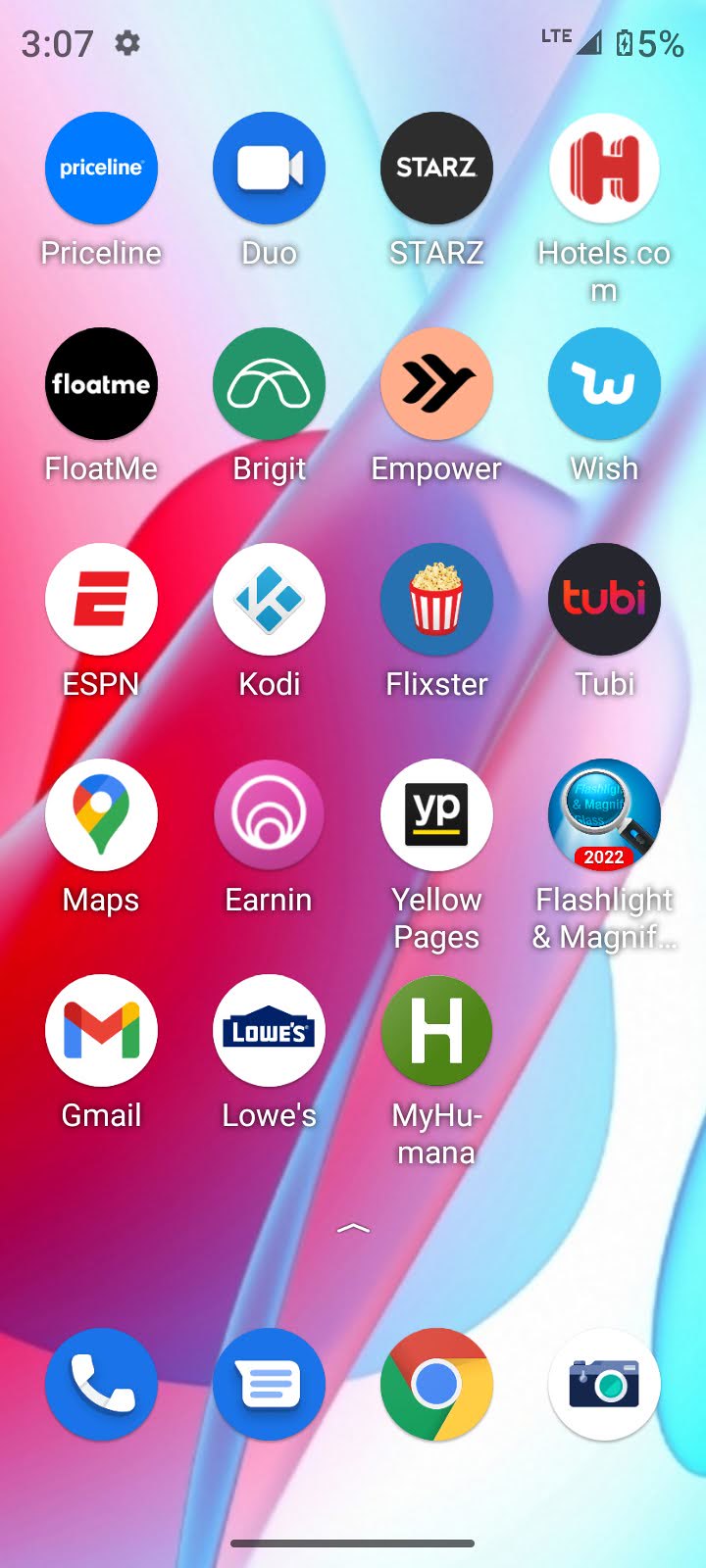This screenshot captures the home screen of an Android smartphone with a colorful, intricately designed background resembling bubbles in shades of red, purple, blue, white, and sky blue. The screen features approximately 23 apps, including Priceline, Duo, Stars, Hotels.com, Floatme, Bridget, Empower, Wish, ESPN, Kodi, Flixster, Tubi, Maps, Ernan, Yellow Pages, Flashlight, Immagnify, Gmail, and Lowe's, along with MyHumana. The bottom of the screen displays four primary icons: Phone, Messages, Google Chrome, and Camera. The phone is connected to the LTE network, showing a battery charge of 5% and the time 3:07. Only the contents of the screen are visible, suggesting a focus on app organization and aesthetic rather than the physical device. The presence of multiple streaming apps like Kodi, Flixster, and Tubi indicates that the user likely enjoys accessing free and potentially pirated TV shows and movies.